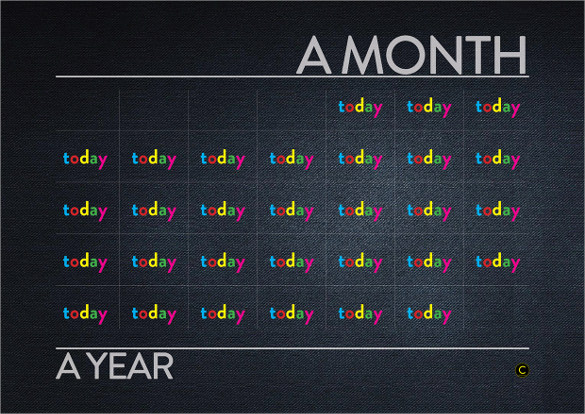The image is a template for a calendar, featuring a grid of rectangles typical of a monthly layout, but with an unconventional twist. Each square in the grid contains the word "today" written in lowercase letters, with each letter in a different color: T in blue, O in red, D in yellow, A in green, and Y in pink. The background resembles dark grey denim fabric, with a subtle, cloth-like texture. At the top right, there is grey text in all-uppercase that reads "A MONTH," accompanied by a thin horizontal grey line extending almost the full width of the image. Similarly, at the bottom left, there’s grey uppercase text stating "A YEAR," with another thin gray line running just above it. The overall design is minimalist yet colorful, with a black-gray gradient framing the edges, and it visually presents an artistic representation of time and daily emphasis.